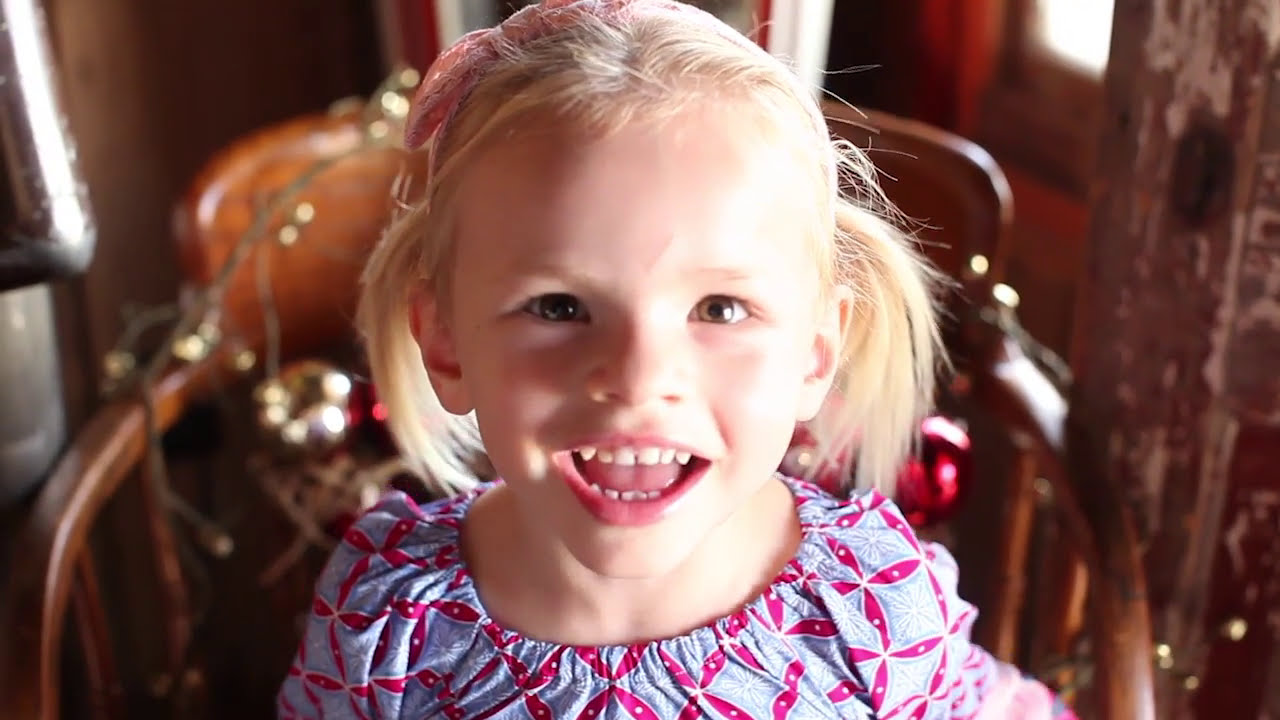In a warmly lit indoor setting, a joyful young girl with blonde pigtails and light skin is sitting on a large, old-fashioned wooden chair adorned with festive Christmas lights and ornaments. Her expressive amber-brown eyes are shining as she looks up at the camera with a wide, open-mouthed smile that reveals her white teeth. She has red lips and small, delicate features, including visible ears, neck, and shoulders. A pink bow accents her hair on the left side. Her outfit features a light blue or gray blouse with a scrunchie neck, decorated with pink flower graphics and white dots on the petals. Behind her, the background includes a blurred scene with a window framed in red, a wooden wall, and various metallic elements. The coziness of the setting, combined with her radiant happiness, makes for a heartwarming portrait.